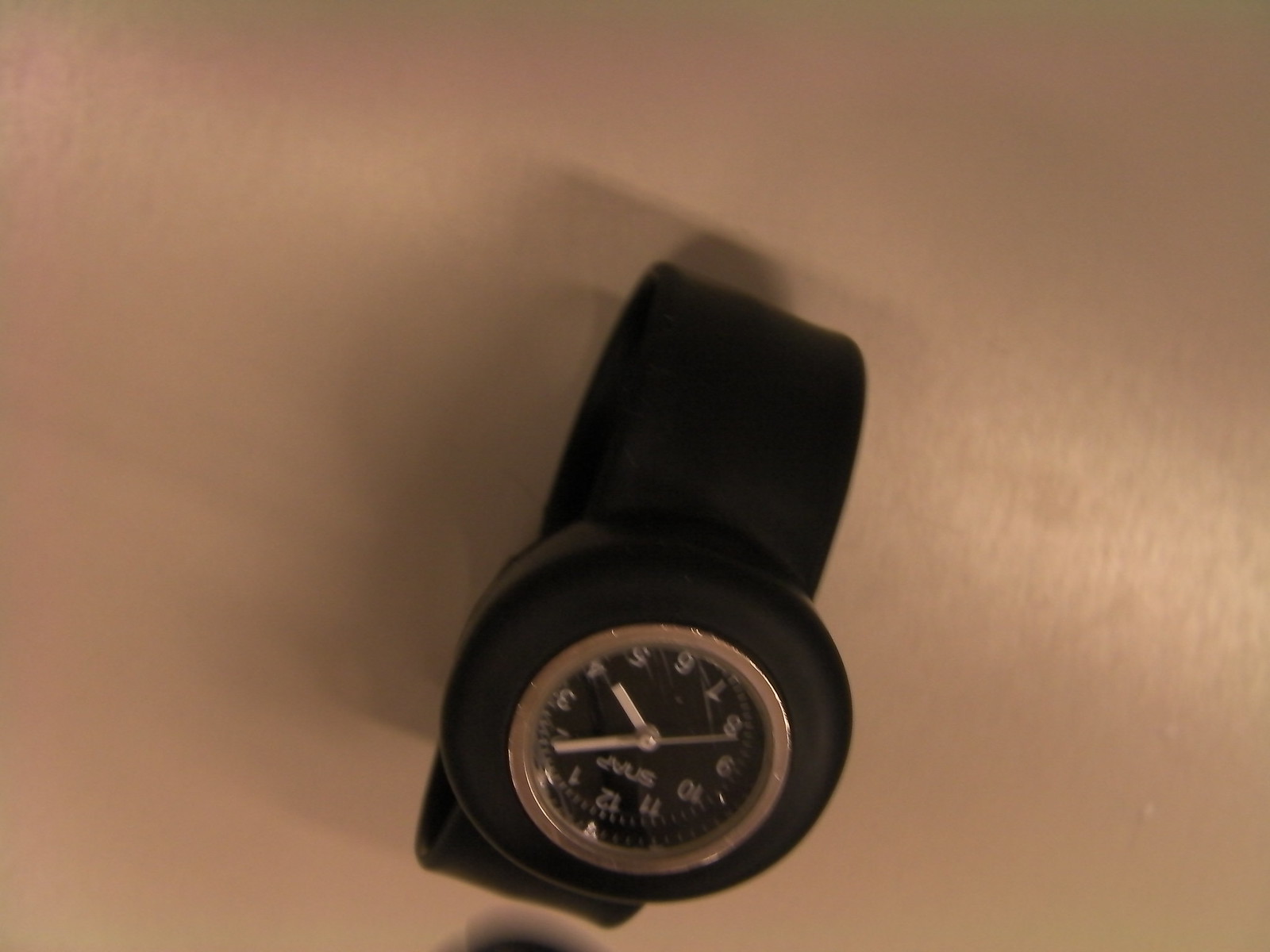This is an upside-down photograph of a black wristwatch situated on a hard, light-colored surface. The wristwatch features a wide black band, which appears to be made of either leather or a nylon material, and forms a circular shape beneath the watch as it would if worn on a wrist. The large black bezel encases the black face of the clock, surrounded by a thin silver rim. The face of the clock is detailed with silver numbers marking the hours, while the hour, minute, and second hands are also silver, with the additional detail of the hour hand pointing at 4, the minute hand at 2, and the second hand at the 8 position. A closer inspection reveals a silver inner circle within the black bezel. The photograph is taken in a low-light setting, casting faint shadows around the watch. Additionally, there is an inscription in white on the clock face—potentially the brand name—which appears to read "SNAP," though it is challenging to decipher clearly due to the orientation.